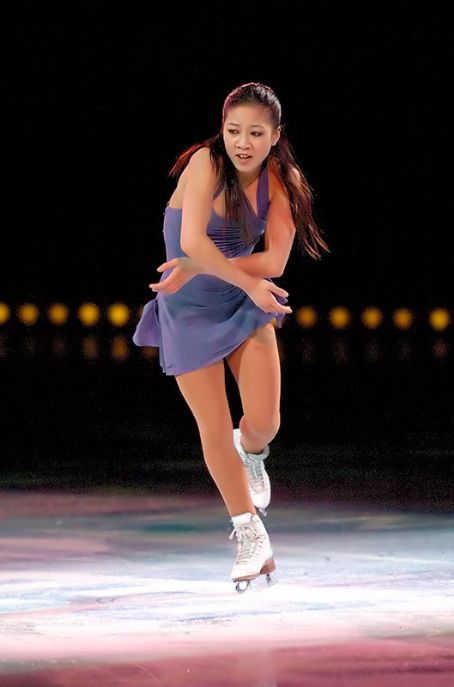The image depicts a professional ice skater of Asian descent, possibly Kristi Yamaguchi or Michelle Kwan, captured mid-performance on an ice rink. She is dressed in a light blue or off-purple halter-top dress, which reveals her skin-colored stockings that extend up to her thighs. She gracefully exhibits her skill, with her long, dark, flowing hair pulled back, and her expressive face slightly open in concentration. The skater's white ice skates glint under the rink's lights, with her right leg extended forward, supporting her weight, while her left leg is slightly bent and lifted. Her arms are crossed in front of her body, indicative of an intricate move, perhaps preparing for or concluding a jump. The rink is bathed in colorful lights, casting shades of pink and green on the white ice, creating a vibrant visual effect. Bright yellow lights form a horizontal row against the otherwise dark background, serving to highlight the dynamic motion and intense focus of the lone skater on the ice.